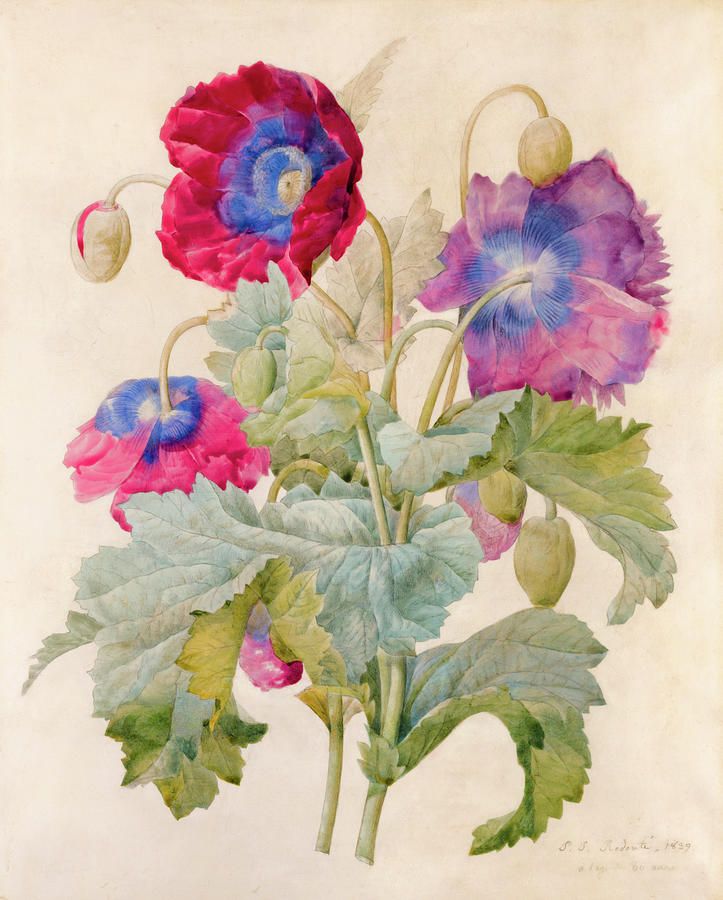This image depicts an artistic painting with a beige background, subtly accented with light brown stains. At the lower right corner, there's an indistinct signature, possibly beginning with "SS." The artwork features a composition of flower stems and large, vibrant flowers with accompanying leaves. At the base, two greenish-brown stems rise, quickly producing leaves that curve downward. These leaves exhibit a gradient with darker greens at the bottom and lighter greens at the top. The stems then extend, curving to the right and left.

On the right, one stem culminates in a large purple flower with a blue center. Above this flower, another stem bears an unopened bud with a tan outer shell. To the left, a prominent red flower with a blue interior and yellow pollen emerges, accompanied by a smaller stem harboring a similarly encased bud with a sliver of red peeking through. Beneath this, there is another red and blue flower, drooping upside down.

Overall, the painting contrasts fully bloomed, colorful flowers with unopened buds, creating a dynamic and vibrant scene against the neutral backdrop.